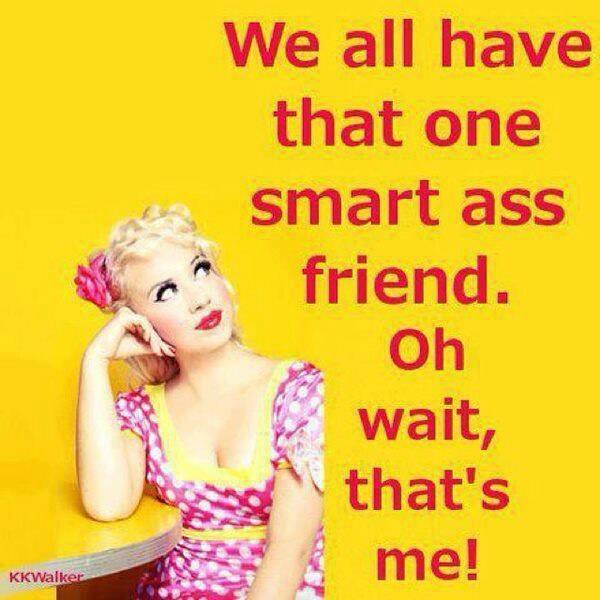The image is an animated yellow poster featuring a woman on the left with striking details and impactful text in red. The woman's blonde hair is adorned with a pink flower, and her vibrant red lips and long eyelashes are distinctly noticeable. She is gazing upward to the right, her head slightly tilted and resting on her left arm, which is supported by her fingers. She wears a u-neck dress that is pink with white polka dots, and yellow accents around the collar and waist.

The red text on the right of the poster reads line by line: "We all have that one smart-ass friend. Oh, wait, that's me. See you next time." 

The woman seems to be leaning on a yellow countertop with grayish sides. At the bottom left corner of the image is the signature "KK Walker" with the initials capitalized. Her right arm is visible up to the elbow but then extends further down out of the image view.